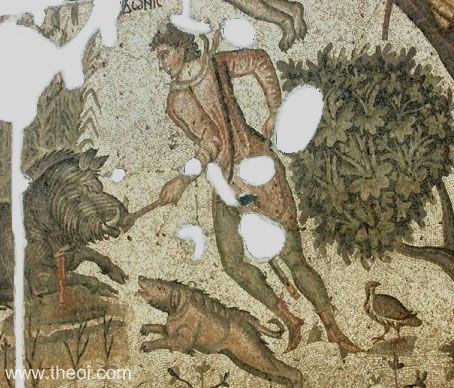This detailed painting, likely AI-generated as suggested by the watermark "www.the.ai.com" in the lower left-hand corner, depicts a dramatic medieval hunting scene. A warrior, dressed in a white long-sleeve coat, green pants, and brown boots, is engaged in combat with a wild boar. The boar, black with fangs protruding from its lower jaw and hair bristling on the back of its head, is being poked in the nose by the warrior's stick. At the warrior's feet, a brown dog with black ruffled fur is lunging at the boar, adding to the chaos of the moment. Behind the hunter, a branch heavily clustered with leaves hangs, possibly the source of the claws suspended above his head. Adding to the forest ambiance, a pheasant or grouse-like bird can be seen standing near the warrior, perched on or near a leaf, looking around alertly. The intricate details and action captured in this piece evoke the intensity and raw struggle of a hunter's life in medieval times.